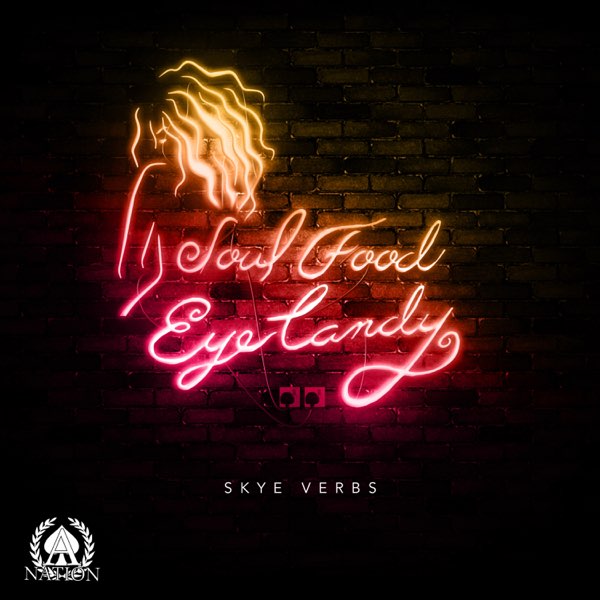The image presents a vibrant and elegant neon sign against a dark background, mounted on a tan brick wall adorned with large decorative patterns. The glowing neon signage reads "Soul Food Eye Candy" in an artistic, cursive font that exudes a feminine touch. At the top left of the sign, wavy lines hint at a depiction of a woman's hair. Beneath the words "Eye Candy," smaller, plain white text spells out "Sky Verbs." Interesting details populate the bottom left corner, where a circular logo reading "A Nation" is encircled by golden wheat stalks that curve gracefully around the letter 'A'. The wall also features a switchboard with visible cords plugged into it. This descriptive scene melds aesthetics of urban street art with hints of digital art representation, creating a visually engaging and multifaceted image.